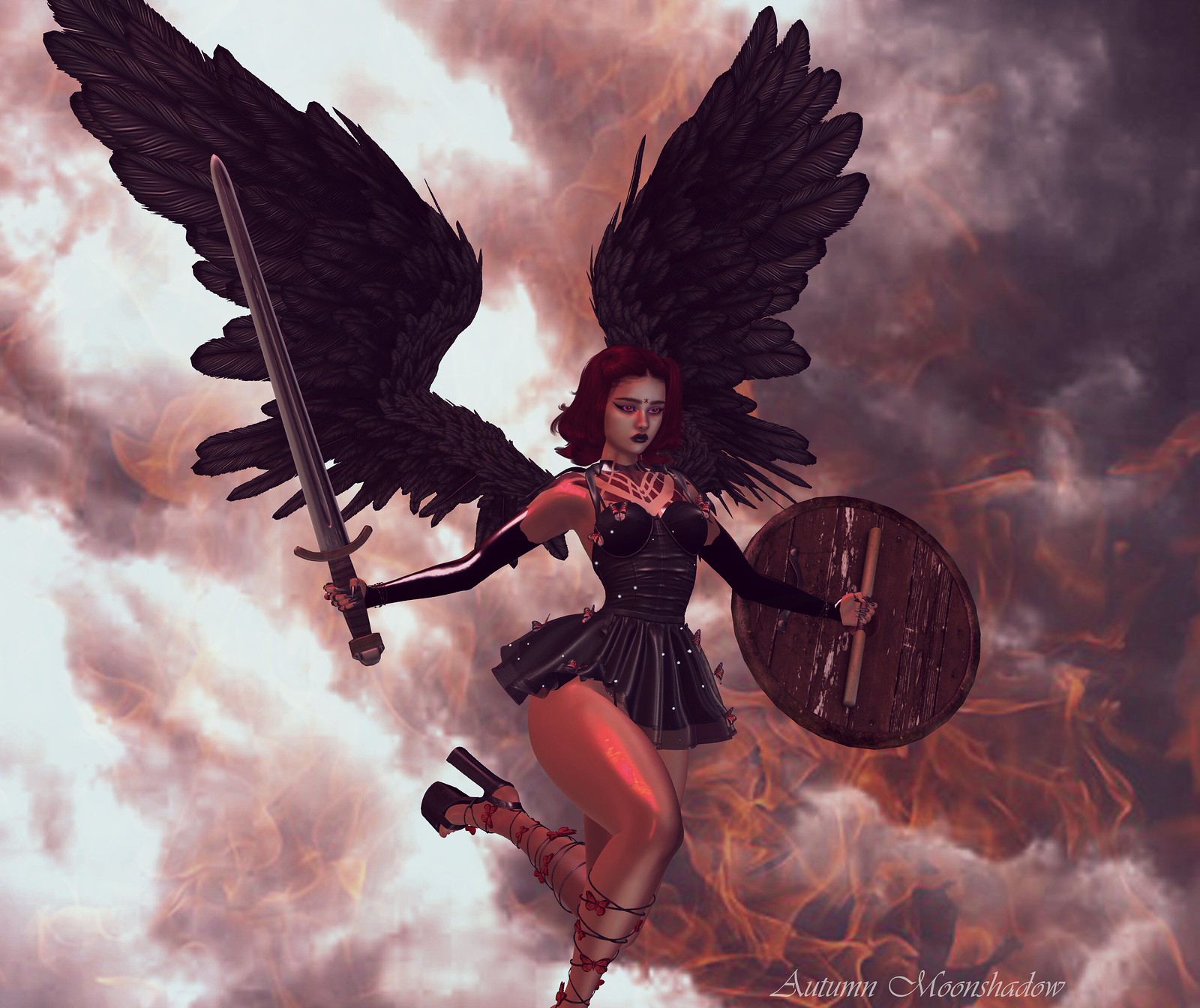This square-format artwork, likely a fantasy illustration, features a dynamic scene with a young woman at its center. Set against a background of mottled clouds and hues of pale orange, pink, and gray, evoking a smoky sky, the female figure stands out dramatically. She is depicted running, with one leg extended behind her, and appears almost to be in flight, characterized by two large black feathered wings emerging from her back. Her dark hair, parted in the middle, frames her face, which is adorned with a black necklace and a bendy on her forehead.

In her left hand, she holds a round shield, possibly wooden, strapped to her arm, while her right hand wields a large, outstretched sword. She is dressed in a very short black dress, complemented by a black corset and black gloves that reach up to her biceps. Her exaggerated, platform high heels feature straps and bows winding around her calves. 

Tattooing is visible around her neck and shoulders, adding to her warrior appearance, and her bare thighs are prominently featured. The overall composition suggests she might be considered a Valkyrie or a warrior fairy. In the lower right-hand corner of the image, the signature "Autumn Moon Shadow" is inscribed in a white script font.